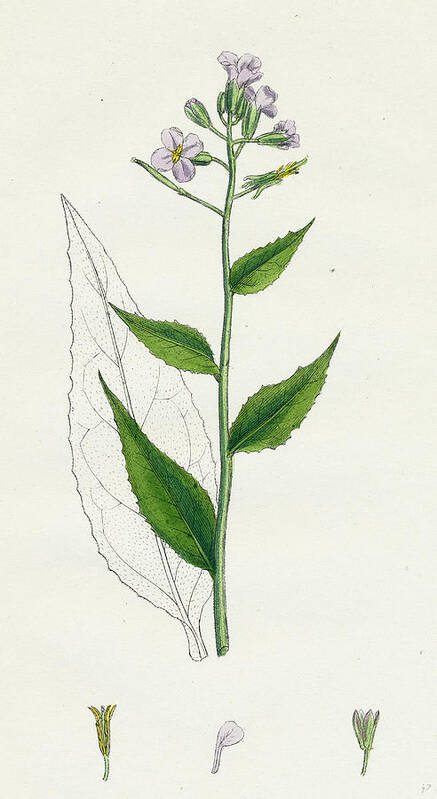This detailed illustration on off-white, possibly tan or cream-colored paper, depicts a botanical sketch of a flowering plant. The plant features a long, green stem adorned with four alternating, serrated-edged leaves that diminish in size from bottom to top. These teardrop-shaped leaves are accurately detailed with a background black-and-white pencil drawing that highlights their vein structure. At the top of the stem, several flower buds are in various stages of blooming, with some still unopened. The blossomed flowers are light lilac or whitish-purple with four petals and yellow centers. At the bottom of the illustration, there are three smaller, detailed sketches: one shows a plant bud with emerging yellow, the second displays a blooming bud starting to reveal its colors, and the third focuses on a single petal. The illustration portrays an antique or classic style, highlighting the plant’s anatomical features with both color and monochrome elements.